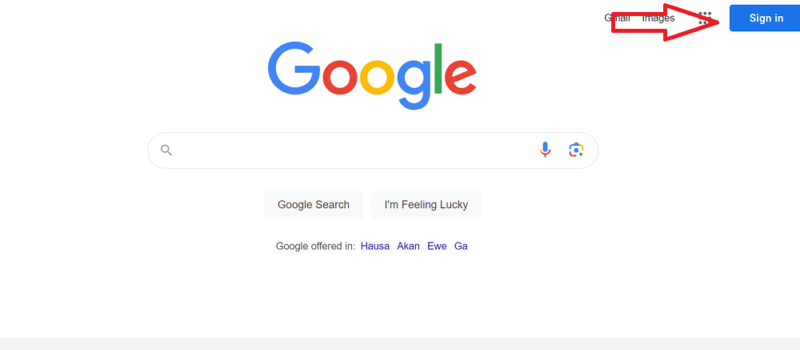The image displays a minimalistic Google search page on a computer monitor with a plain white background. In the top right corner, there is a blue rectangle featuring white text that reads "Sign In." Next to it, in black text, are the words "Gmail" and "Images," accompanied by an icon consisting of nine gray dots arranged in a 3x3 grid. Superimposed over this section is a prominent, bold red arrow pointing directly to the "Sign In" button.

Slightly left of center is the iconic multicolored Google logo, comprising a blue "G," red "O," yellow "O," blue "G," green "L," and red "E." Directly below the logo is the search bar, which includes a small microphone and camera icon on its far right. Beneath the search bar are two light gray buttons; the left one is labeled "Google Search," and the right one says "I'm Feeling Lucky." Below these buttons, the text indicates that Google is offered in Hausa, Akan, Ewe, and Ga.